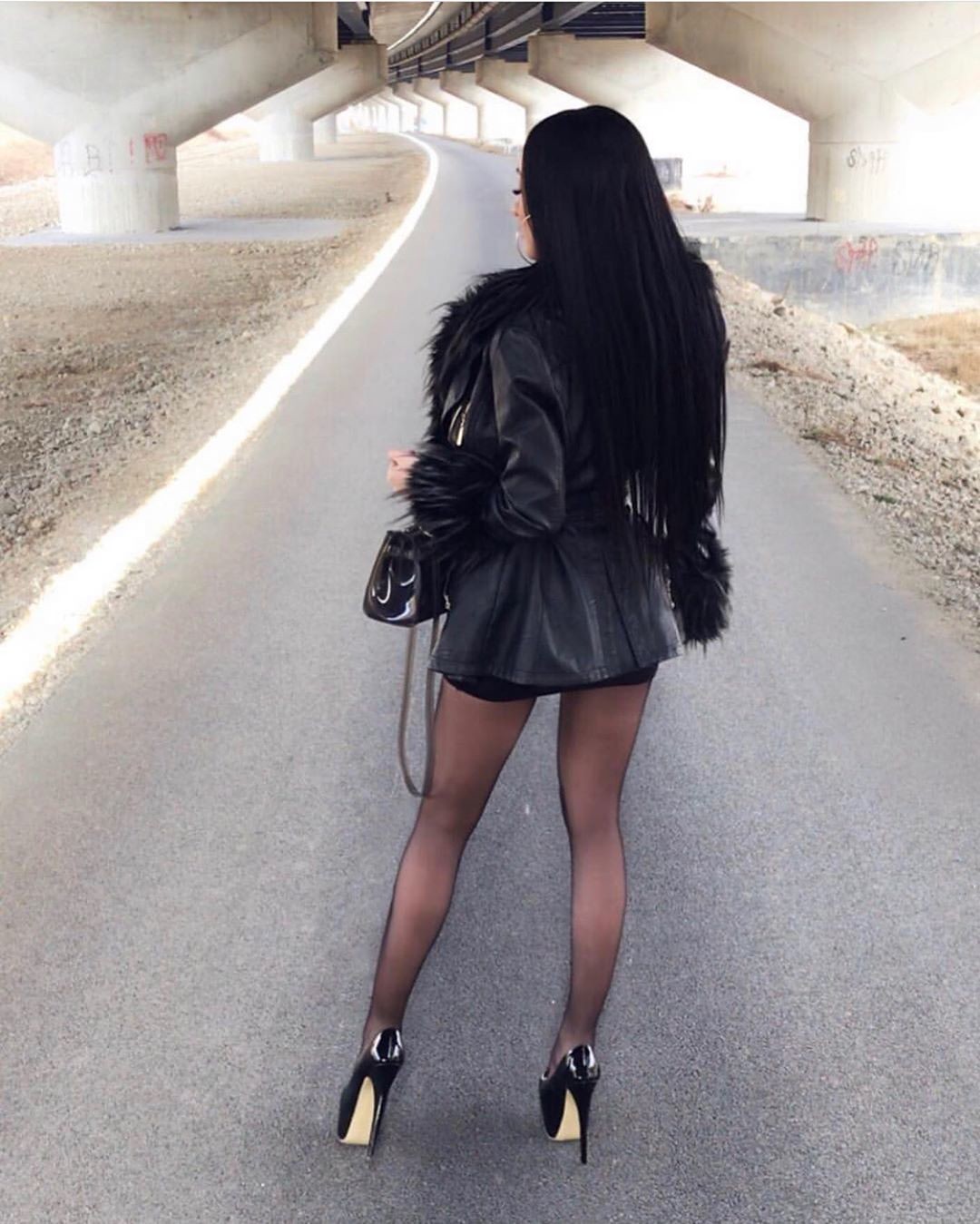In this detailed image, a woman with long black hair is centrally positioned, standing on a paved asphalt road, likely a bike or walking path, that extends straight up through the center of the frame. The setting is under the overhang of an elevated highway or train track, characterized by large concrete supports that recede into the distance. The road features a white line on the left side and is flanked by gravel, dirt, and rocky hills on both sides.

The woman is dressed in a black leather jacket with feathery or furry wrist and lapel details, a short black skirt, black stockings, and black high heels. She carries a small black purse. The overall color palette of the image includes shades of gray, tan, brown, black, white, and red, suggesting a midday, outdoor setting. The backdrop includes the underside of the overpass or bridge structure, adding to the symmetrical and somewhat gritty urban atmosphere of the photo.